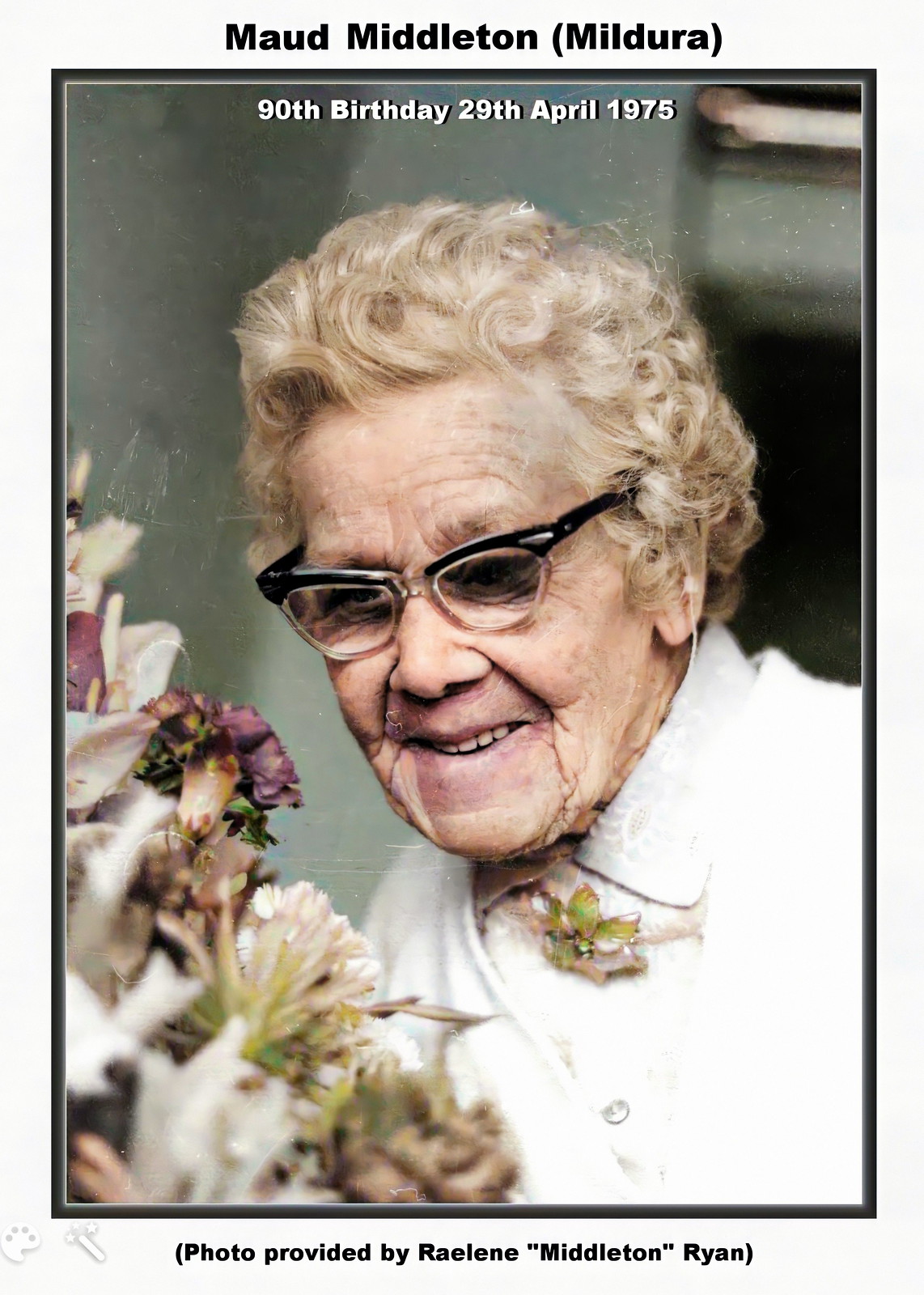This image is a detailed black-and-white photograph of an elderly Caucasian woman identified as Maud Middleton, with "Mildura" in parentheses above the frame. The inscriptions state it is her "90th birthday, 29th April 1975." Maud, who has curly, blondish-gray hair and wears horn-rimmed glasses, is smiling faintly and appears elegantly dressed for this special occasion in a white blouse, a white sweater, and a necklace that rests just under her blouse's collar. She leans forward slightly, gazing down at a floral bouquet comprising carnations, roses, and lilies, situated in the lower left quadrant and slightly out of focus, enhancing the intimate moment captured. The plain gray wall in the background ensures all attention is on Maud and the bouquet. Below the photograph, it mentions, "photo provided by Raylene Middleton Ryan," framing the image with a black border to highlight it further.